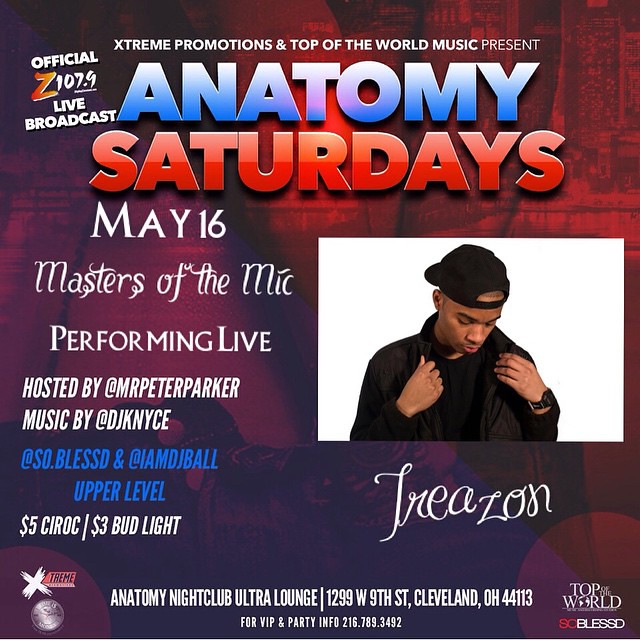In this vibrant, multi-colored event poster, predominantly featuring purple and red hues, the central focus is a photo of a young black man wearing a black hoodie, a backwards black baseball cap, and a black watch. He appears to be adjusting his jacket while looking down. The image is set against a white background on the right side of the poster. 

The top section prominently announces the event with "Official Z107.9 Live Broadcast," "Extreme Promotions," and "Top of the World Music Present" in white lettering. Beneath this, in a white-to-blue gradient, is "Anatomy" followed by "Saturdays" in a pink-to-red gradient. Further details reveal the event date, "May 16th," and highlight it as “Masters of the Mic Performing Live,” hosted by mr. Peter Parker. Music will be provided by DJ KNYCE (@DJ KNYCE), So Blessed (@So.Blessed), and I Am DJ Ball (@I am DJ Ball). 

Lower on the poster, the image of the man is captioned with his stage name, "Trezon (T-R-E-A-Z-O-N)," in white lettering. Adjacent to this, the flyer advertises drink specials including $5 Ciroc and $3 Bud Light. 

Additional information includes venue details that read "Anatomy Nightclub Ultra Lounge, 1299 West 9th Street, Cleveland, Ohio, 44113," and a contact number for VIP and party info: 216-789-3492. The "Extreme" logo is featured in the lower left-hand corner, and the "Top of the World, SC Blessed" logo is in the lower right-hand corner.